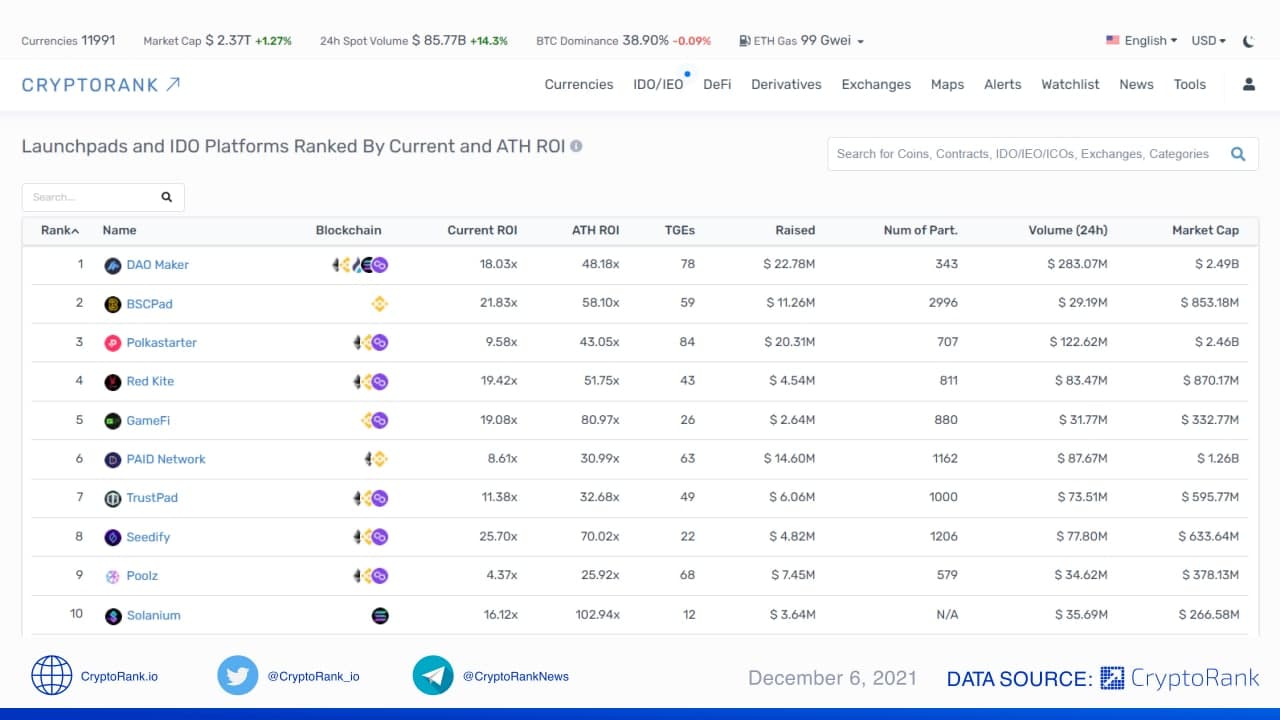This is a screenshot of a website page featuring a comprehensive summary of cryptocurrency market data. The header is white with various sections of information from left to right. Beginning with "Currencies," it lists 11,991 in dark grey text. Following a spacing, it displays "Market Cap" at $2.37 trillion, highlighted by smaller green numerals indicating a +1.27% change. Further right, "24-Hour Spot Volume" or "24H" is noted with $85.77 billion in larger dark grey text, alongside green numerals showing a +14.3% change.

Next, "BTC Dominance" is reported at 38.90% in dark grey text, with smaller red numerals indicating a -0.09% change. A dark grey gas pump icon marks the section for ETH gas prices, listed as 99 GWEI (capital G-W-E-I) in dark grey text. A grey triangle pointing down follows.

To the far right, there is an American flag followed by a dropdown menu label "English" and another dropdown for "USD," both with triangles pointing down. This section is accompanied by a dark grey icon of a crescent moon. A thin light grey line separates this header from another white header below.

Within the second header, on the left, there is blue all-caps text reading "CRYPTO RANK," accented by an arrow pointing up and to the right at a 45-degree angle. The rest of the header features significant negative space with more medium grey text on the right. The layout is clean and structured, allowing for quick access to critical cryptocurrency market metrics.